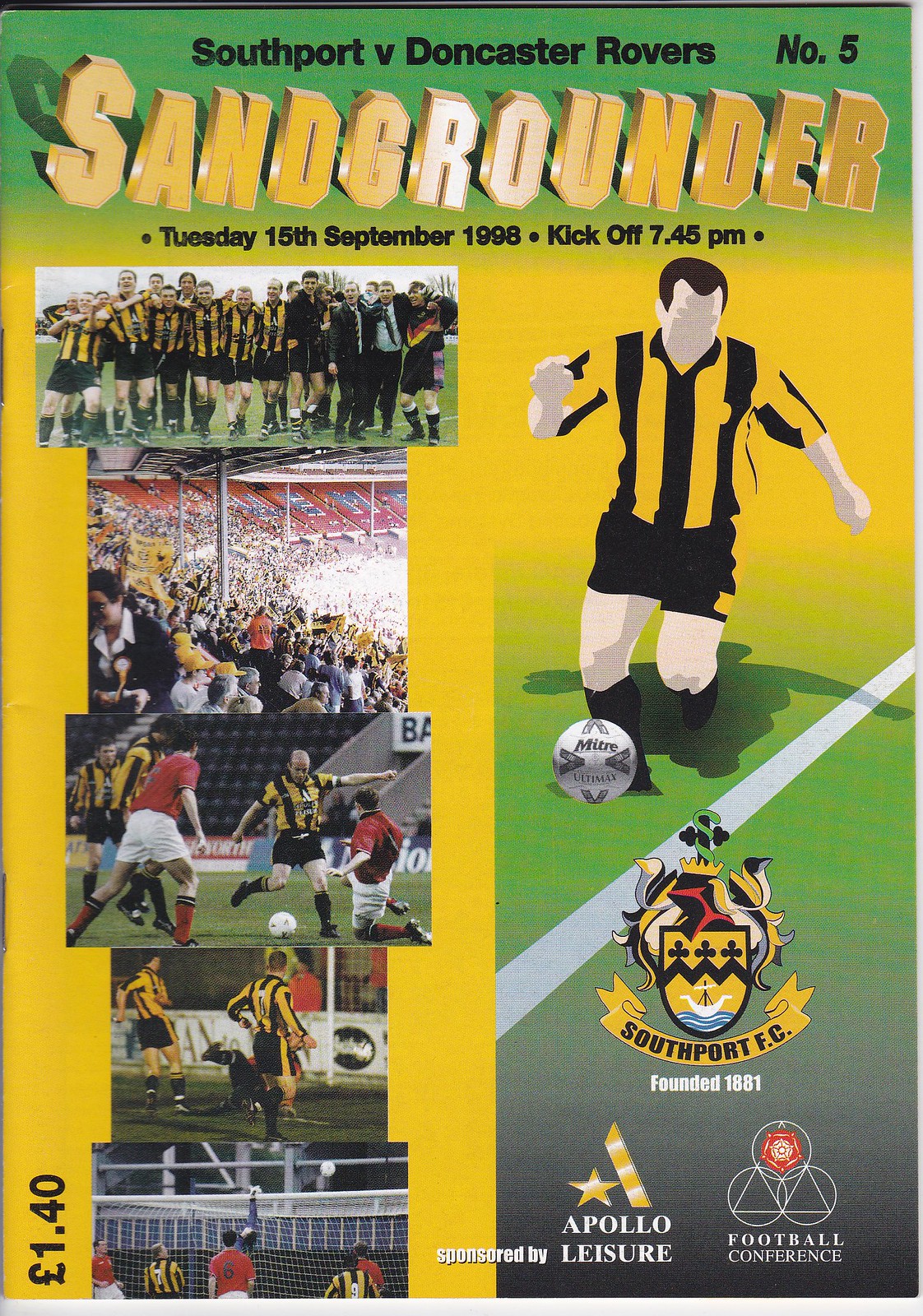The advertisement flyer is for an exciting football match featuring Southport vs. Doncaster Rovers, taking place on Tuesday, September 15th, 1998, with a kickoff at 7:45 PM. The title "Sand Grounder" is prominently displayed at the top, indicating the event or tournament's name.

The vibrant background is a blend of green and yellow, with an animated image of a soccer player in black and yellow apparel on the right side, standing on a green field marked by a white stripe. Beneath this animated player are three significant insignias representing the soccer league and affiliated organizations. These include a logo for Apollo Leisure, the Football Conference, and the crest of Southport FC, established in 1881.

On the left side of the flyer are various photos from previous sporting events or earlier in the season, showcasing players in action, fans in the crowd, and team photos. Among these images are scenes of players kicking the soccer ball into the net, and group shots of players in red and white attire. The flyer is full of energy and excitement, capturing the anticipation for the upcoming game.